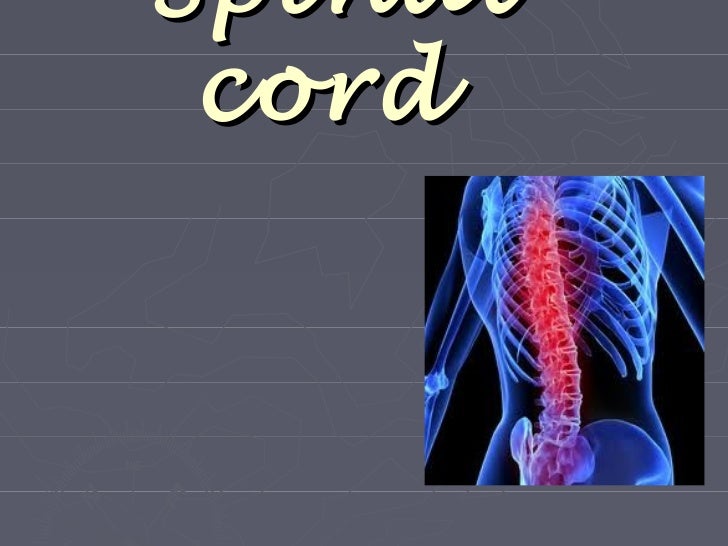This image, resembling a slide from a textbook or PowerPoint presentation, features a gray background with a pattern of thin white and light gray horizontal lines. In the bottom right corner, there is a digital x-ray image of a human body, showcasing transparent blue bones that reveal the ribs, arms, upper pelvis, and particularly the spinal cord. The spinal cord is highlighted in red, which, when combined with the blue of the bones, creates a purple hue near the spine. At the top of the slide, there is partially visible cursive text in light yellow with black shading, where the word "cord" is readable, and "spinal" is likely the obscured portion. The composition includes elements commonly found in educational slideshows, with a focus on the anatomical depiction of the spine.